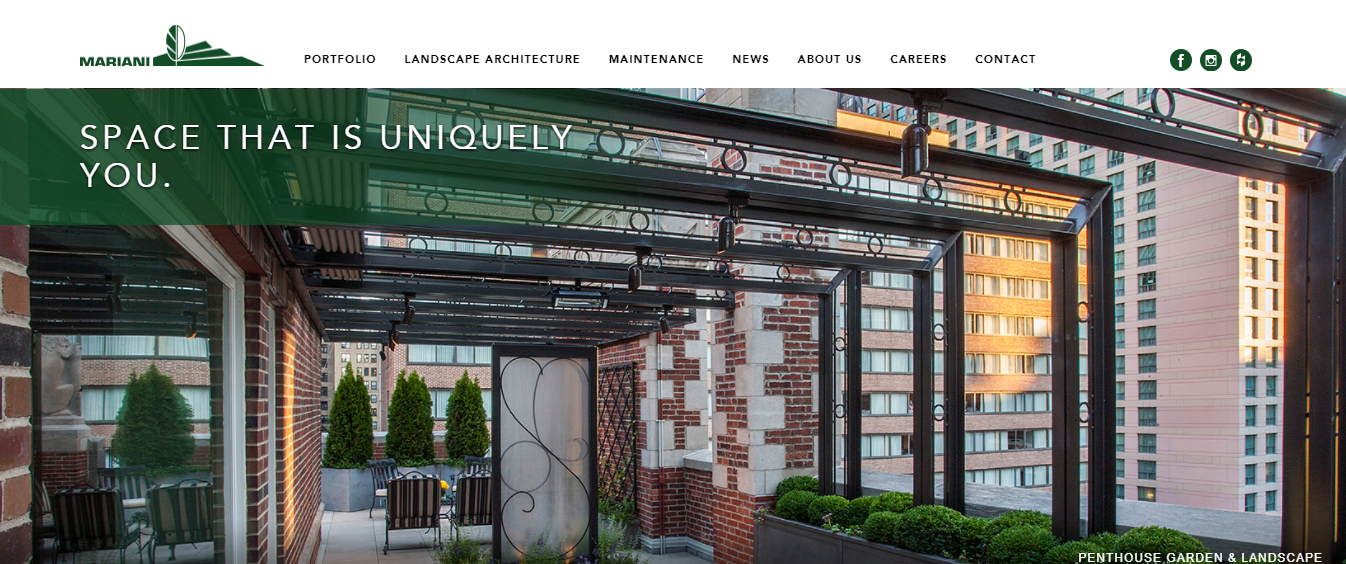This image depicts the homepage of the Mariani website. At the top of the page, there is a white background featuring the Mariani logo. The logo consists of the word "Mariani" in green text accompanied by a centrally positioned leaf icon that is half green and half white. Adjacent to the logo, there is a navigation menu with tabs labeled "Portfolio," "Landscape Architecture," "Maintenance," "News," "About Us," "Careers," and "Contact." To the far right of the navigation menu, there are icons representing links to social media pages.

Below the header, the main image showcases a rooftop space designed for outdoor dining. The area is adorned with plants and trees and offers a scenic view of surrounding buildings on the right. In the bottom right corner of this image, text reads "Penthouse Garden and Landscape." Additionally, in the upper left corner, there is a green box with white text that says "Space That Is Uniquely You," emphasizing the personalized approach to their landscape designs.